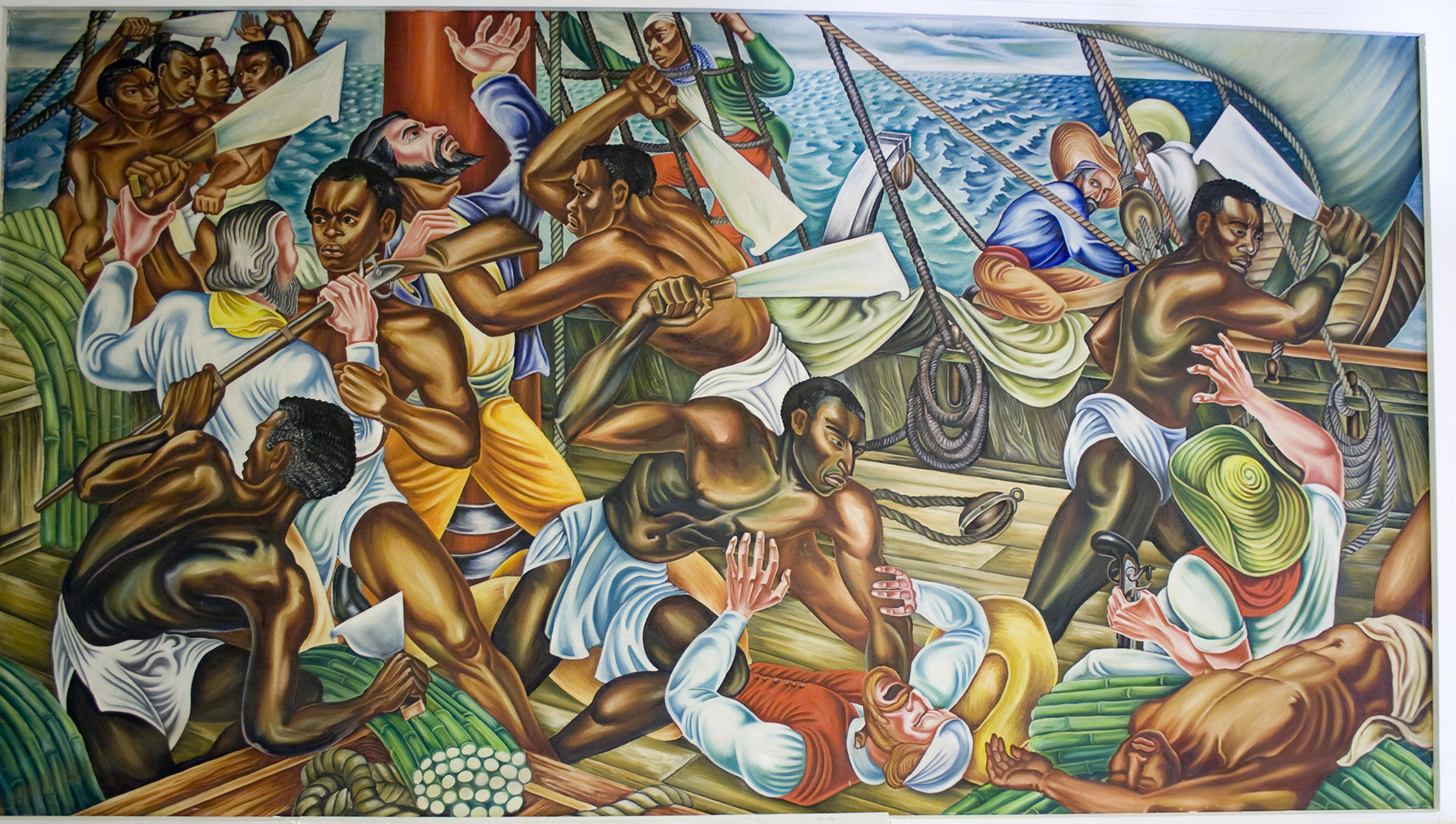This detailed, hand-drawn artwork, displayed as though it is within a game, captures the intense moment of a slave uprising aboard a ship in the middle of the ocean. The scene, vividly illustrated in a mural style, relays the chaos and determination of the enslaved individuals as they revolt against their captors. In the center of the piece, a slave, distinguishable by his red hat and minimal clothing, is seen pinning down a white man, presumably a captain given his long sleeves and uniform, preparing to strike with a large machete. Around them, other slaves are fiercely fighting back; some wield machetes while others grapple with their oppressors. One can observe a slave handler attempting to escape into a lifeboat in the background. Despite several white captors being armed, their guns and knives seem ineffective against the unyielding revolt. The ocean waves in the background enhance the stark contrast between the ship’s turmoil and the vast, indifferent sea surrounding it. The intricate and colorful details of the clothing, expressions, and weaponry heighten the dramatic and dynamic nature of this uprising scene.